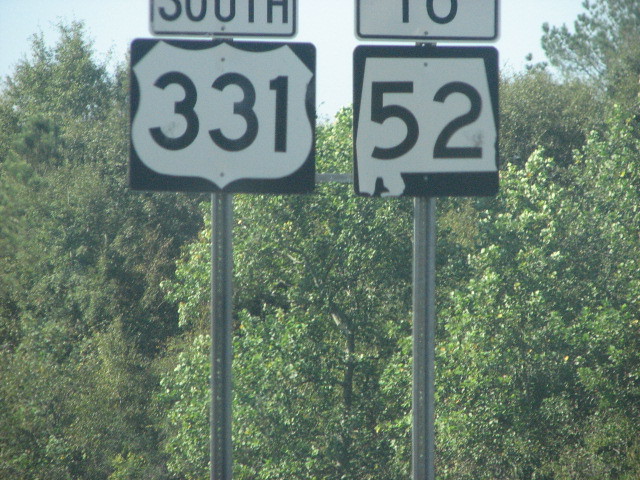Two highway signs stand side-by-side against a lush backdrop of deciduous trees on a clear day. The trees display a diverse palette of greens, ranging from light pastel to vibrant grass and deep forest hues. Above the foliage, the sky peeks through in a light blue shade accentuated with fluffy white clouds. 

In the foreground, the highway signs are mounted on tall, slender metal poles. The sign on the right comprises two parts: a smaller rectangular sign at the top with a white background and black text reading "South," and below it, a larger square sign featuring the number "331" in black. The sign on the left displays two numbers: "2" at the top and "52" beneath it, both in black text.